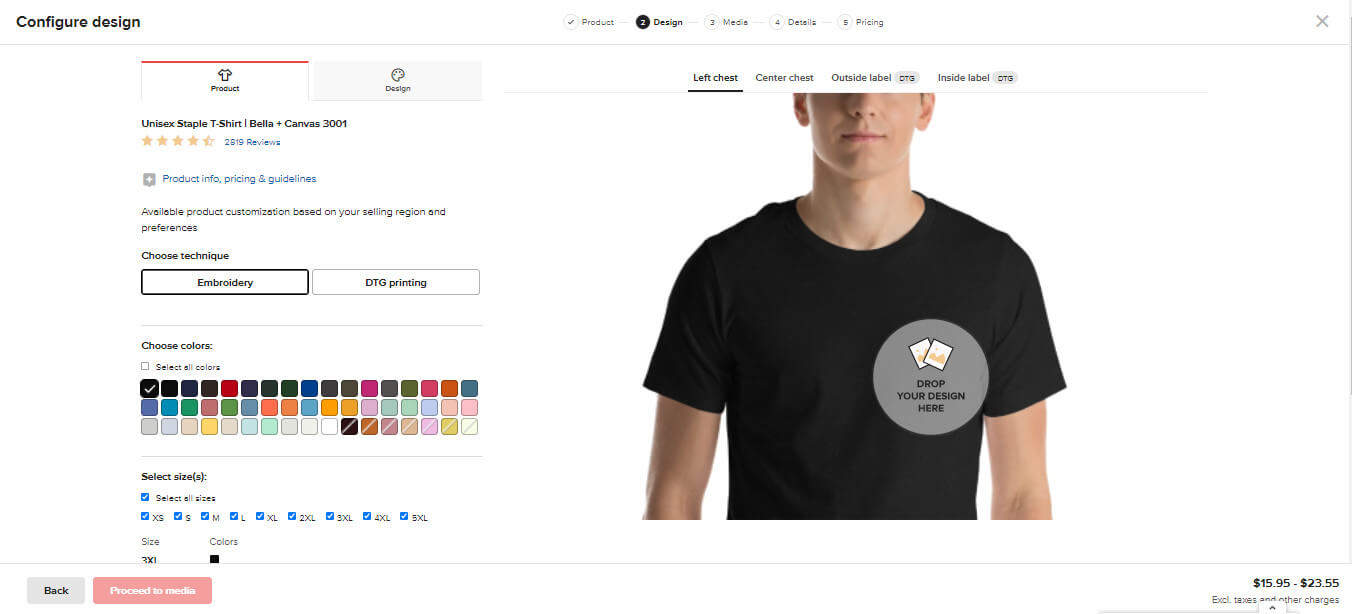This screenshot is taken from a website that allows users to design their own custom t-shirts. In the top left corner of the screen, there's a label that reads "Configure Design." Centrally positioned at the top are navigational tabs labeled "Product," "Design," "Media," "Details," and "Pricing." In the top right corner, an 'X' button is visible for closing the interface.

Dominating the middle section is an image featuring a man wearing a black t-shirt inscribed with the placeholder text, "Drop Your Design Here," indicating where users can visualize their custom designs. 

On the left side of the screen, there’s a detailed section catering to customization options. It specifies that the type of shirt available for customization is a unisex staple t-shirt, Bella + Canvas 3001, detailed with 2,119 reviews. The section also includes tabs for product information, pricing, and guidelines, as well as customization options tailored to the user's selling region and preferences. Additionally, users can choose between embroidery or printing techniques and select from various color options.